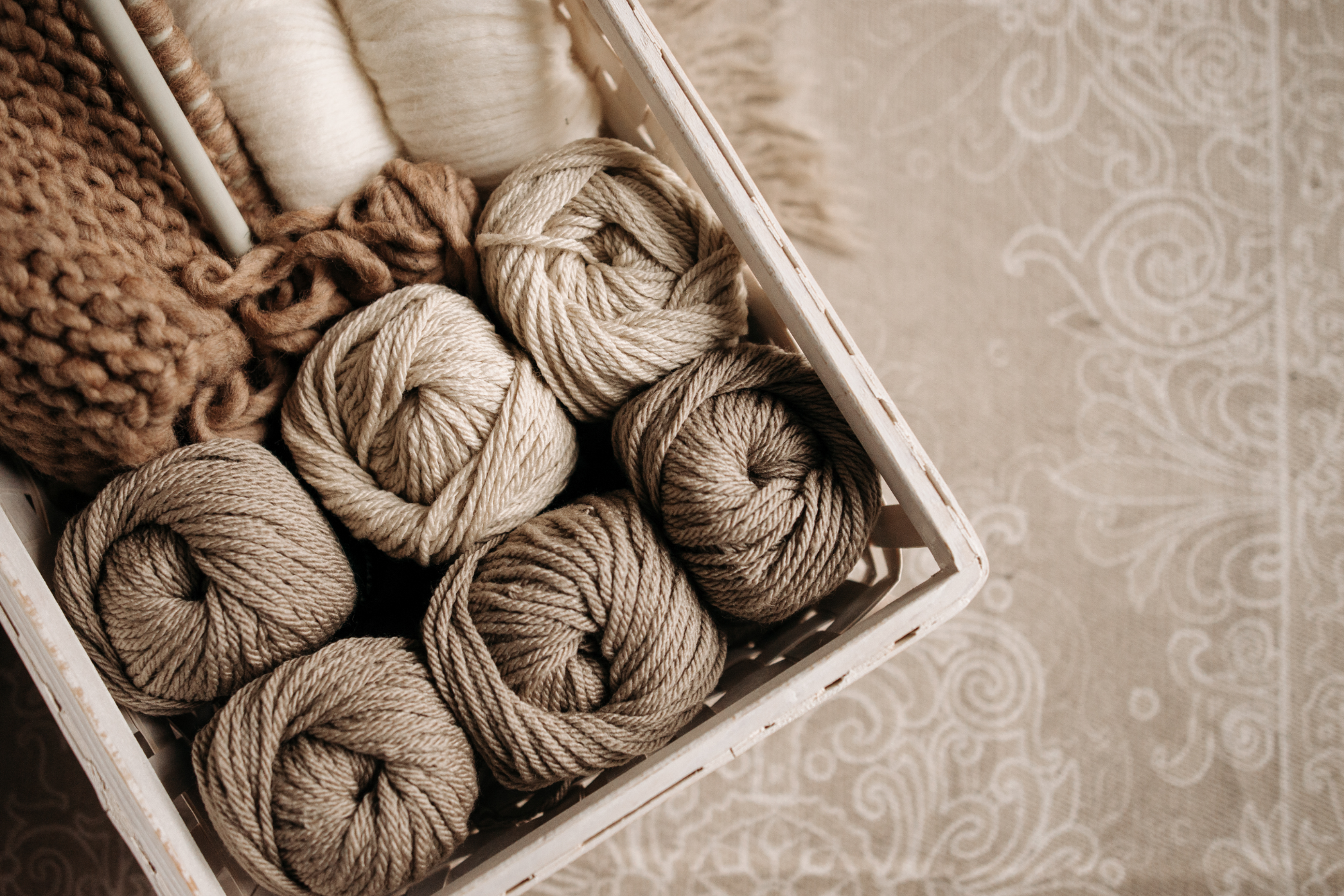This overhead photograph features a white crate partially visible, containing six bundles of yarn in varying shades of white, tan, and brown. In the upper left corner of the crate, a brown knit item is in progress. To the right of the yarn, there are white, linen-like fabric pieces. The crate rests on a light grayish-tan linen tablecloth adorned with an interwoven design of white circles, floral motifs, leaves, and swirls. Tucked in the upper left corner is a glimpse of a white cylindrical object, possibly a crocheting needle.